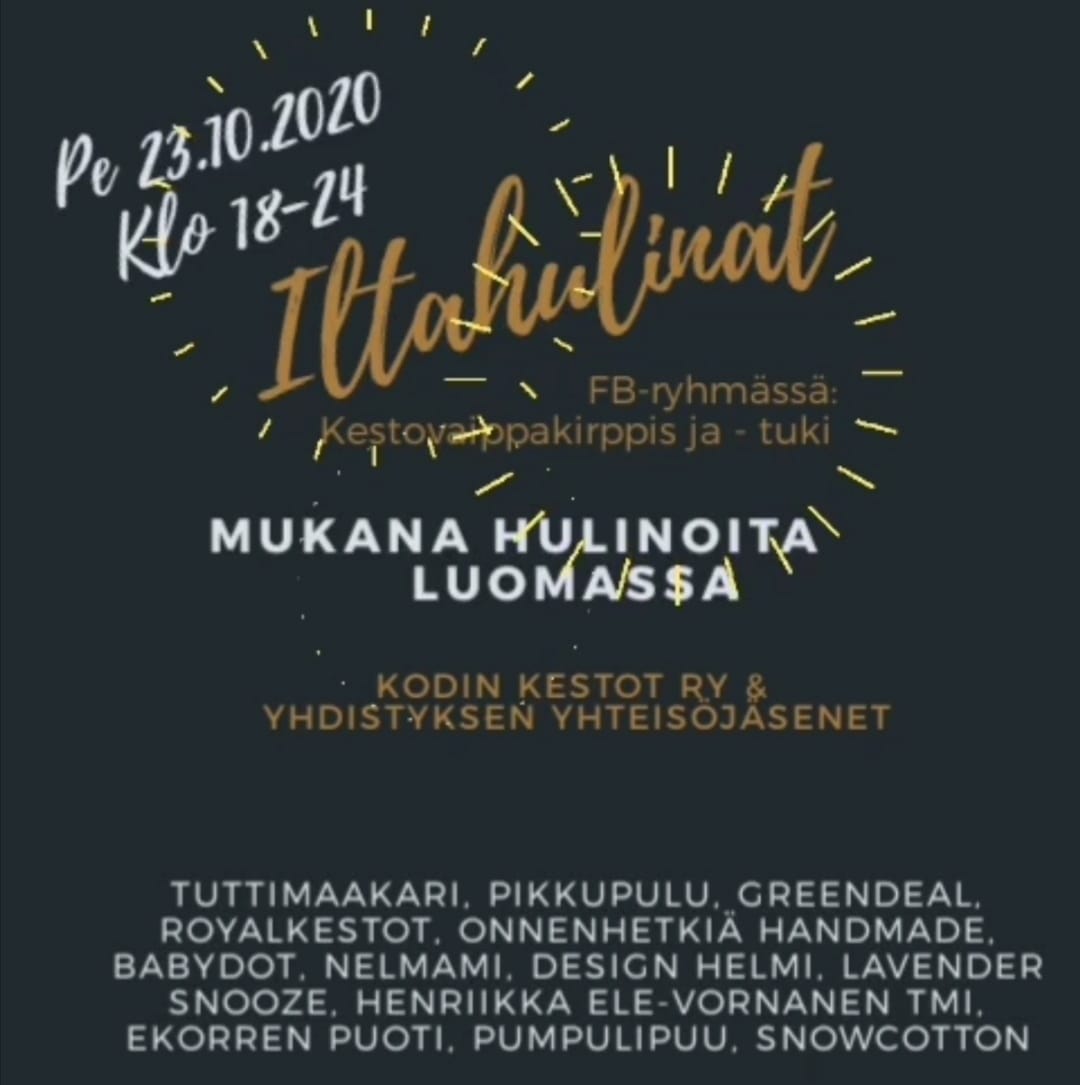This image features a sign or advertisement, predominantly in a non-English language. In the upper left-hand corner, the text reads "P.E. 23.10.2020 K.L.O. 1824." Below this, the word "Iltu Hulunat" is displayed in gold letters. Following this, there is a section of text also in gold, though the language is not specified. Underneath the gold text, bolded white letters in all capital letters stand out prominently. Further below, a second set of words in gold appears. At the very bottom of the image, additional white text is present, most of which is in a non-English language. However, there are a few recognizable English words: "handmade baby, dot design, lavender, snooze, and snow cotton."